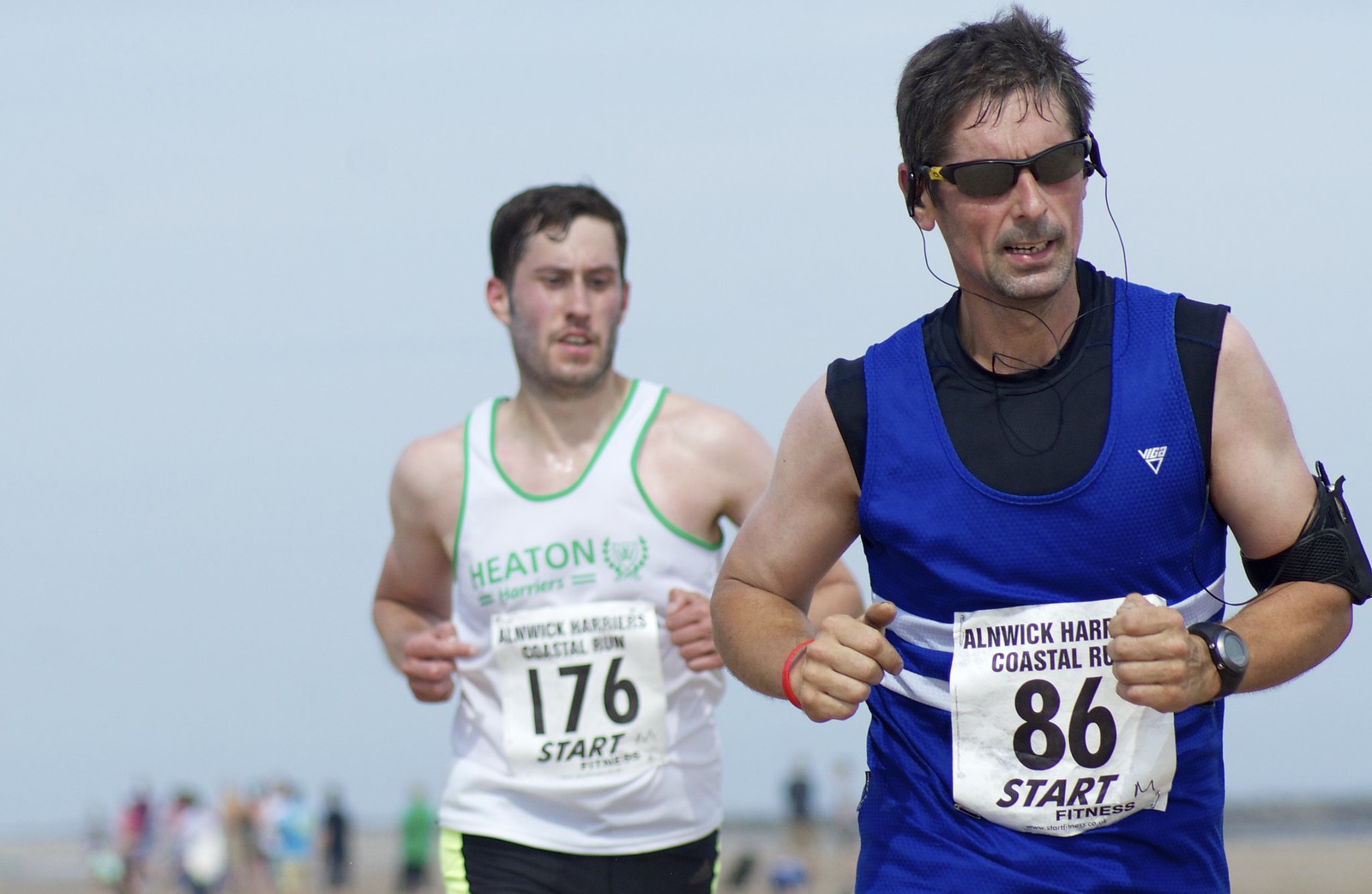This photograph captures two men engaged in a marathon, set against a light blue sky with blurred spectators in the distant background. The main focus is on these two runners. The man on the right, who is slightly ahead, is adorned in a dark blue tank top over a black undershirt and is equipped with glasses, earphones, and an elbow pad. His race number, 86, is prominently displayed on a label that reads "Alnick Coastal Run" and "Start Fitness." To his left, a little behind, is another runner donning a white tank top with green trim, marked with the race number 176, also labeled "Start Fitness." The runners' faces and upper bodies are clearly visible, highlighting their intense focus and effort in the race.